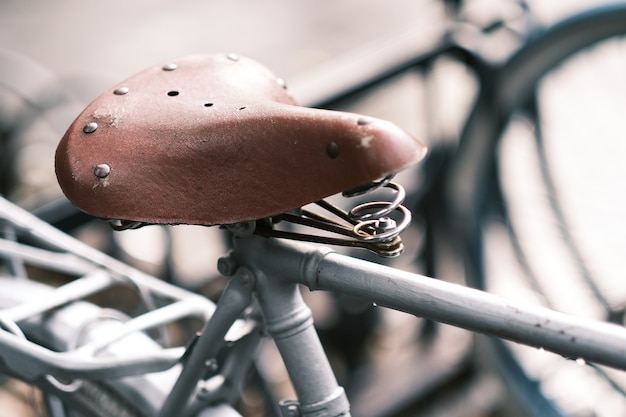The image is a detailed, close-up photograph of a vintage, weathered bicycle seat. The seat itself is a brownish-red leather, adorned with silver rivets both at the back and front, and appears well-worn, lending it an antique look. Beneath the seat, a silver spring is visible, indicating the traditional mounting mechanism. The bicycle frame, which is silver or chrome, extends diagonally from the middle to the right side of the image, while another bar slopes downward to connect with the rear wheel. Behind the seat, there is a fender covering a portion of the back wheel, along with a rack intended for carrying groceries or cargo. The background is blurred, but you can faintly discern the outline of another bicycle, suggesting a setting by a bike rack, possibly on an urban street.